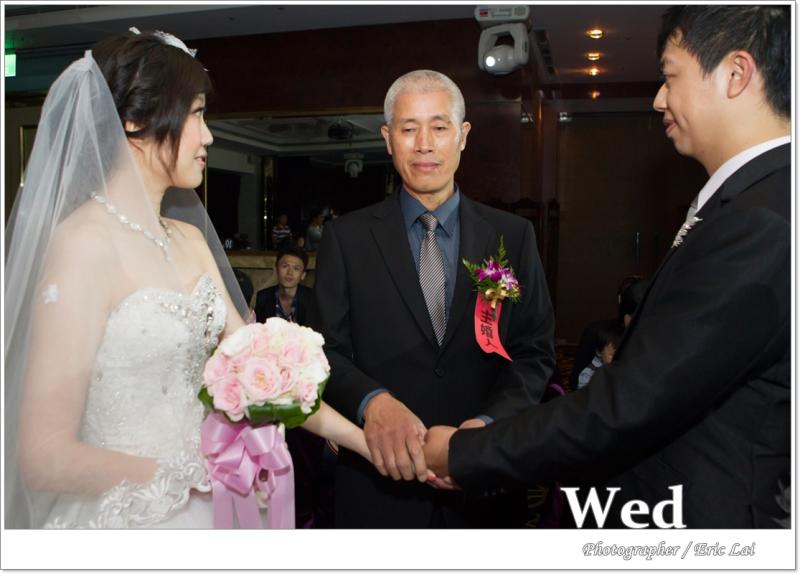In the image, we see a wedding ceremony in progress set against a plain brown wall in a modest room. At the center, an older Asian officiant with short gray hair, dressed in a black suit, a blue collared shirt, and a gray tie, is conducting the ceremony. A large boutonniere adorns his left lapel. The officiant holds the left hand of the bride and the right hand of the groom, symbolizing their union. To the left stands the bride, an Asian woman with short black hair peeking out from under a transparent white veil. She wears a strapless white wedding gown adorned with intricate embroidery, along with a white pearl necklace. Her right hand, bent at the elbow, clasps a bouquet of pink and white roses tied with a pink ribbon. To the officiant’s right stands the groom, also Asian, shown in profile. He has short black hair and wears a black suit paired with a white collared shirt. His left hand is extended forward, holding his bride's hand as they both face the officiant. There is a discernible text at the bottom right corner of the image reading "wed," with smaller italicized text below it indicating the photographer's name, which is challenging to decipher. The backdrop includes a light fixture above the officiant and hints of other elements like a person seated in the background.